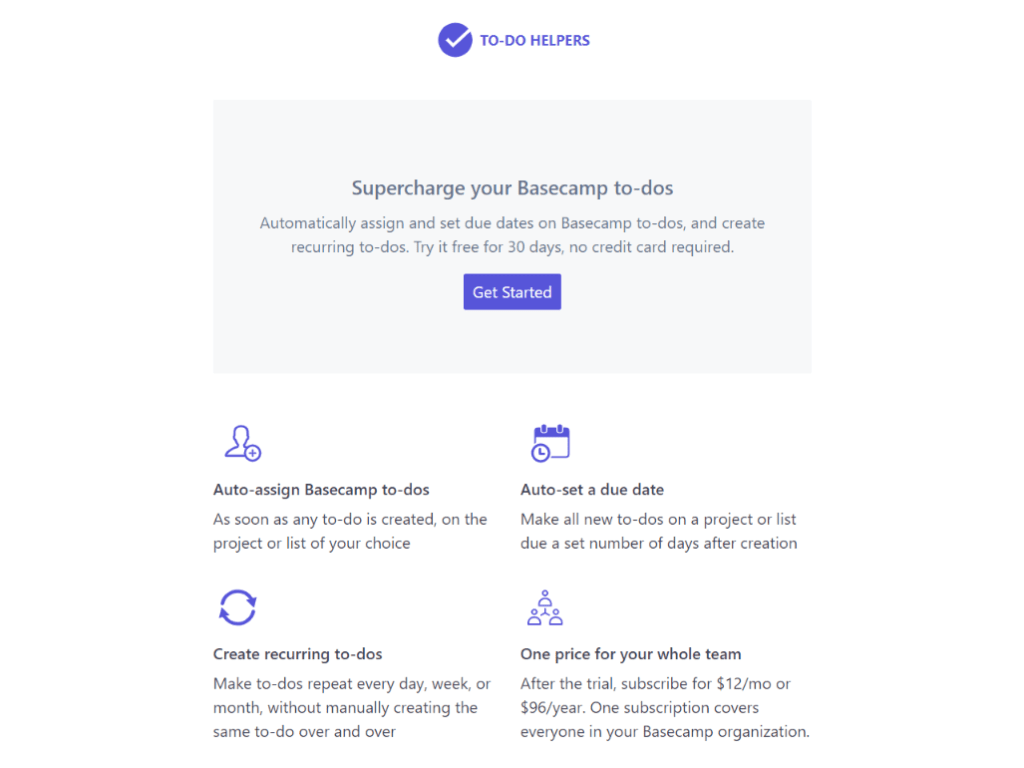The image depicts a web page for a service named "ToDoHelpers". At the top of the page, the heading "ToDoHelpers" is prominently displayed in purple, accompanied by a small checkmark icon encircled in purple on its left side.

Beneath the heading, there is a window with a light grey background containing darker grey text. The main text reads, "Supercharge your Basecamp ToDos." Below, in a smaller font, the text states, "Automatically assign and set due dates on Basecamp ToDos and create recurring ToDos. Try it free for 30 days, no credit card required." Below this text, a purple button labeled "Get Started" is positioned after some space.

Further down the page, aligned side by side, are four feature descriptions, each with an accompanying icon. 

1. The first feature, "Auto-assign Basecamp ToDos," is detailed alongside an icon of a small calendar and timer. The description reads, "Automatically assign ToDos to team members as soon as they are created in the project or list of your choice."
   
2. The second feature, "Auto-set a due date," includes its description and an icon depicting a small calendar with a timer. It reads, "Make all new ToDos on a project or list due a set number of days after their creation."
   
3. The third feature, "Creating recurring ToDos," features an icon of two arrows forming a circle. The text explains, "Make ToDos repeat every day, week, or month without manually creating the same ToDo over and over."

4. The fourth and final feature, "One price for your whole team," is accompanied by an icon of three connected people. It reads, "After the trial, subscribe for $12 a month or $96 a year. One subscription covers everyone in your Basecamp organization."

This detailed and organized layout aims to clearly communicate the functionalities and benefits of using ToDoHelpers.